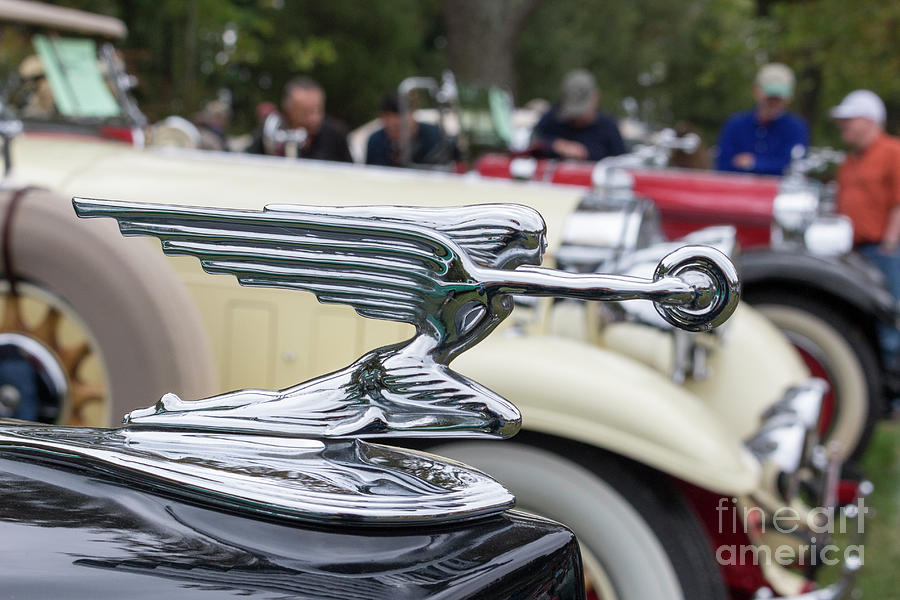This photograph captures a close-up of a chrome hood ornament on the sleek, black hood of an old-time car, highlighted with a Fine Art America watermark in the bottom right corner. The ornament is a highly stylized, silver figure of a woman with streaming hair and outstretched wings, depicting motion as she leans forward, holding a wheel in her extended arms. The detail extends to her dress, which ripples over her legs, with her right knee bent forward and her left leg stretched straight back as if bracing against the wind. In the dim background, a yellow car and a red car, each bearing similar vintage hood ornaments, are visible along with several blurry figures, likely attendees at an antique car show admiring the cars. The overall scene exudes a sense of nostalgia and admiration for classic automotive design.